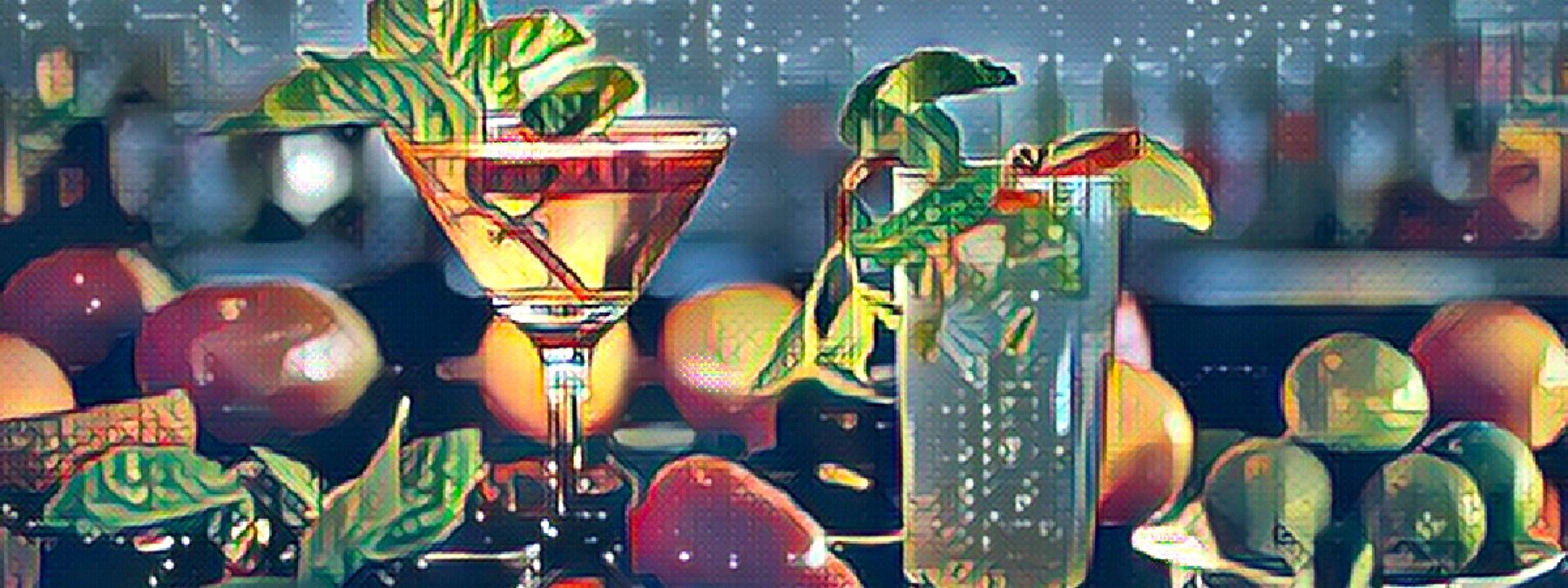The image is a digital, pixelated illustration with a 16-bit style, featuring a detailed depiction of a bar top adorned with various fruits and drinks. Dominating the center are two distinct beverages: on the left, a martini glass filled to the brim with a yellowish liquid, accentuated by a small branch bearing four leaves. To the right, a tall, narrow glass contains a clear liquid, garnished with a slice of lime and sprigs of greenery cascading down the sides. Scattered around the two drinks are pixelated fruits, including mangoes and kiwis, as well as green leaves. The bar top itself is laden with these vibrant fruits, highlighting the image's use of bright shades of green, orange, dark red, and yellow. The background behind the bar is blurry, featuring a white-speckled, grayish texture that adds depth to the scene, complemented by hints of a blue sky with stars. A bowl of limes and other orange and reddish fruits can be discerned in the backdrop, enhancing the overall composition with their vivid colors and abstract representation.